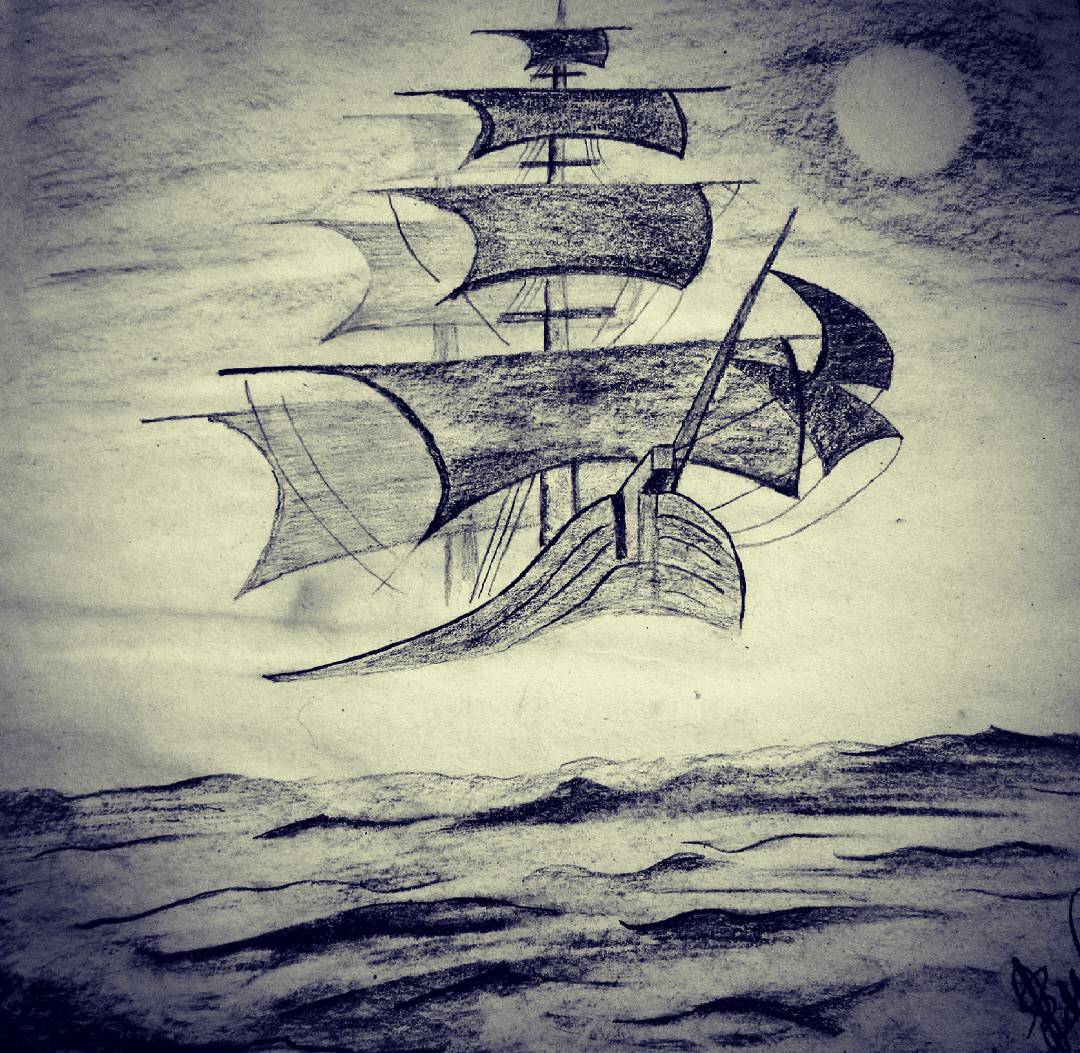In this detailed charcoal drawing on beige paper, an old wooden sailing ship is depicted with meticulous attention to shading and texture. The vessel, which stands roughly eight inches tall, is only partially shown, with the bottom of the ship missing, creating a striking gap between the ship and the wavy ocean below. The wooden hull is rendered in shades of black and gray, capturing the worn texture of the wood. The ship features two tall masts, each with four rectangular sails decreasing in size from bottom to top, and a sharp-pointed bow. Smaller, kite-shaped sails are positioned at the front. The water beneath is illustrated with sharp, dark lines and shaded areas, accentuating the movement of the waves. In the upper right corner, a shaded circle, likely representing the moon or sun, is surrounded by dark clouds, adding a dramatic contrast to the scene. The sky also includes areas of white shading, enhancing the atmospheric depth of the image.